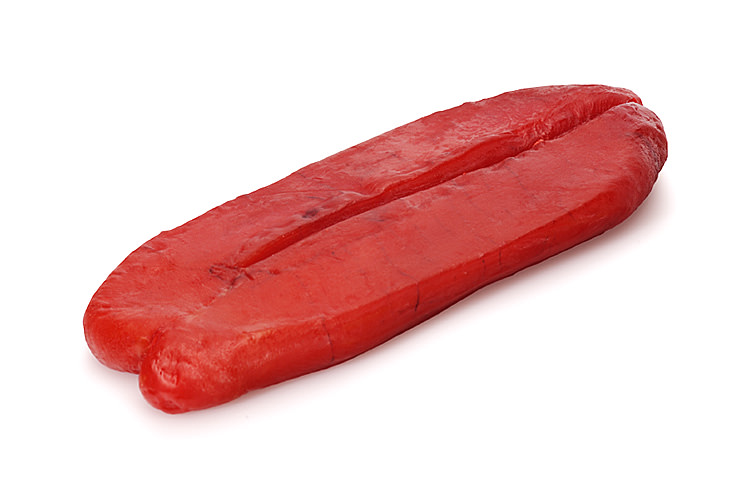This image depicts a reddish-brown object resembling a hot dog or sausage, cut in half and lying diagonally from the lower left to the upper right on a white surface. The object features a seam running down its middle, beginning just below the edge on the left side and continuing to the right, indicating it might be a single item partially split open. The ends of the object are slightly crinkled and appear to be attached at the lower end. The surface has a shiny, seared look, with some black streaks adding to the impression of grill marks. The empty background and lighting suggest an indoor setup. Overall, the object’s texture and color might lead one to believe it to be a cut and grilled piece of sausage rather than a vegetable.